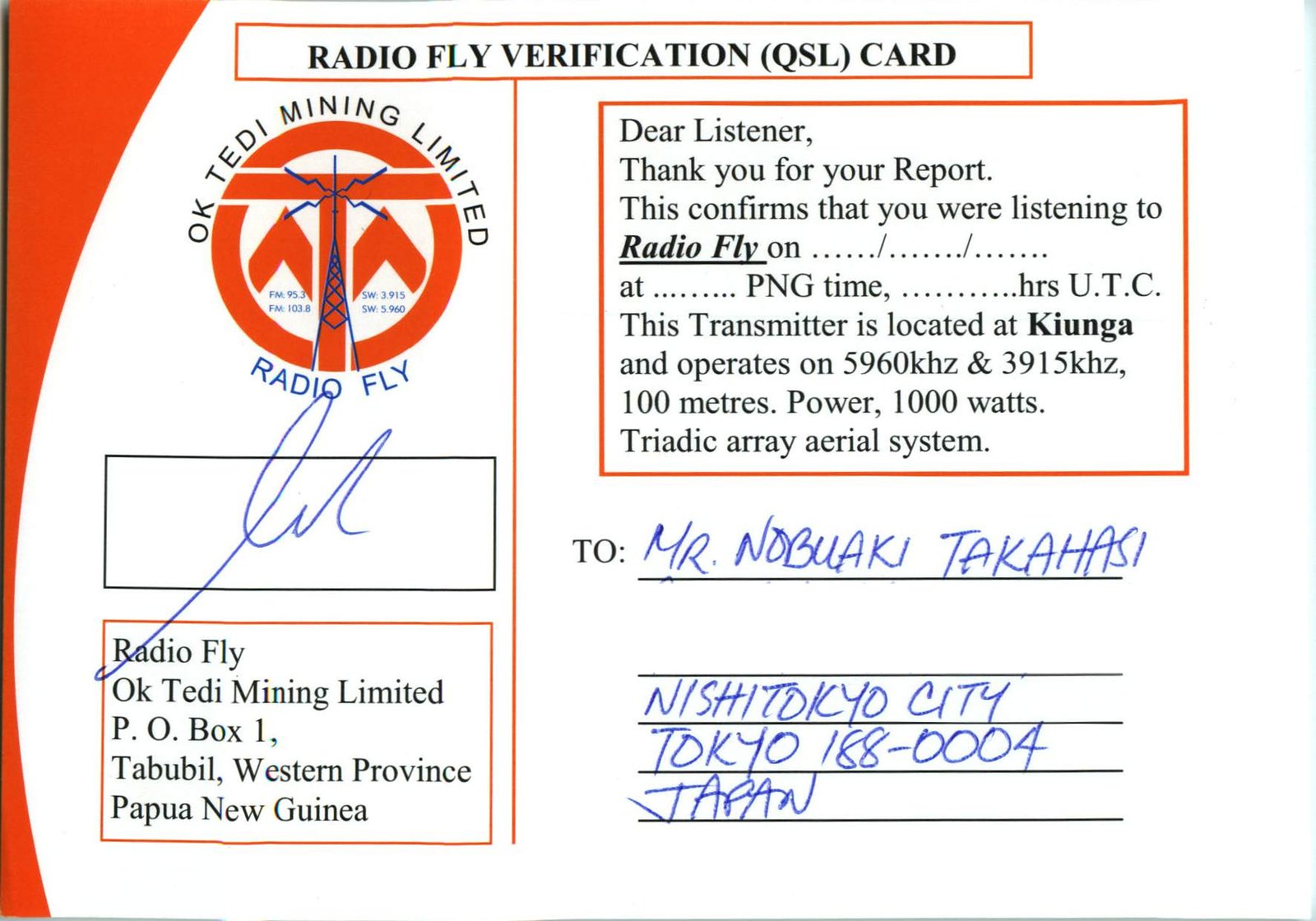The image depicts a detailed RadioFly Verification QSL Card. The card is primarily white with an orange curve on the far left side. At the top, spanning both sections of the card, it reads "RadioFly Verification QSL Card." On the left side of the card, below the top header, is a logo featuring a radio antenna within a circle, surrounded by the text "OK Teddy Mining Limited RadioFly." Below the logo, there is a box with an illegible signature followed by the address: "RadioFly, OK Teddy Mining Limited, P.O. Box 1, Tabubil, Western Province, Papua New Guinea."

The right side of the card contains a message beginning with "Dear Listener," which states: "Thank you for your report. This confirms that you were listening to RadioFly on [blank] at [blank] PNG time, [blank] hours UTC. This transmitter, located at Kayunga, operates on 5960 kHz and 3915 kHz, 100 meters power, 1000 watts, triadic array aerial system." At the bottom of this section is the recipient's address: "To Mr. Nobuaki Takahashi, Nishitokyo City, Tokyo 188-88004, Japan."

The card also features red borders around various text boxes, adding to its structured and informative layout.